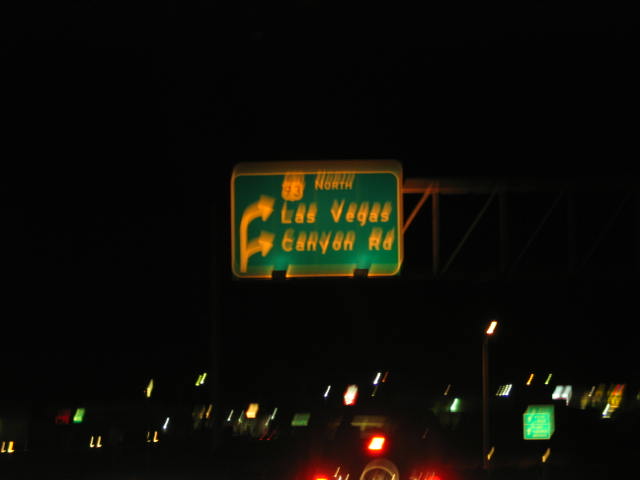In this nighttime photograph, the sky is completely enveloped in darkness. At the center, there's an illuminated traffic sign with a golden edge and golden lettering, likely accentuated by the surrounding lighting. The sign features two distinct lines of text: "93 North" prominently displayed on top, followed by "Las Vegas" and "Canyon Road," both accompanied by arrows pointing to the right. Two lights at the bottom frame the sign, casting a spotlight effect.

Below the main sign, the image fades into further darkness. Scattered throughout this lower portion are various sources of artificial light, notably a series of street lights positioned at higher elevations along the road. Additionally, a green sign is faintly visible in the distance, appearing to be another traffic marker.

Near the bottom section of the image, possibly amidst the scattered lights, is the rear view of a vehicle discerned by three distinct red lights; one situated at the top center and two positioned on each side, likely indicating the tail and brake lights. The scene also captures a few more green lights dispersed along the roadway, contributing to the dimly lit nocturnal ambiance.